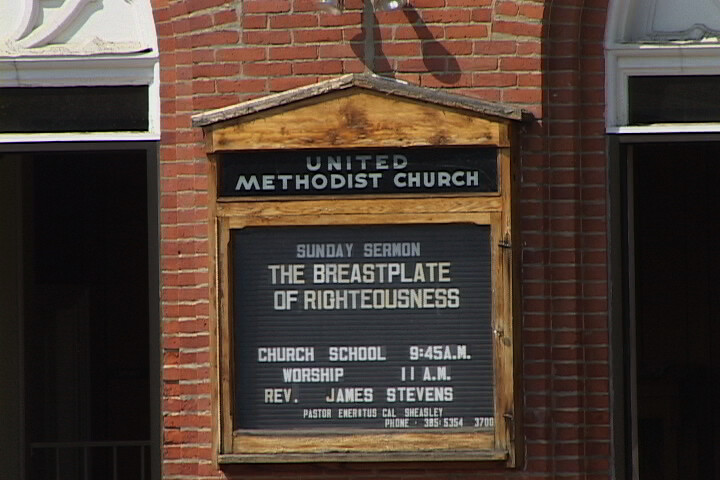The image shows the front of a red brick church building with white moldings above partially visible windows on either side of the structure. Mounted on the central red brick wall is a small wooden sign with a decorative roof. The sign features white lettering on a black background. Across the top, it reads "United Methodist Church," followed by the schedule and details: "Sunday Sermon: The Breastplate of Righteousness," "Church School: 9:45 AM," "Worship: 11 AM," "Reverend James Stevens," "Pastor Emeritus Kel Sheasley," and a contact number, "385-5354." On either side of the sign, there are two open doorways with patches of white above them.